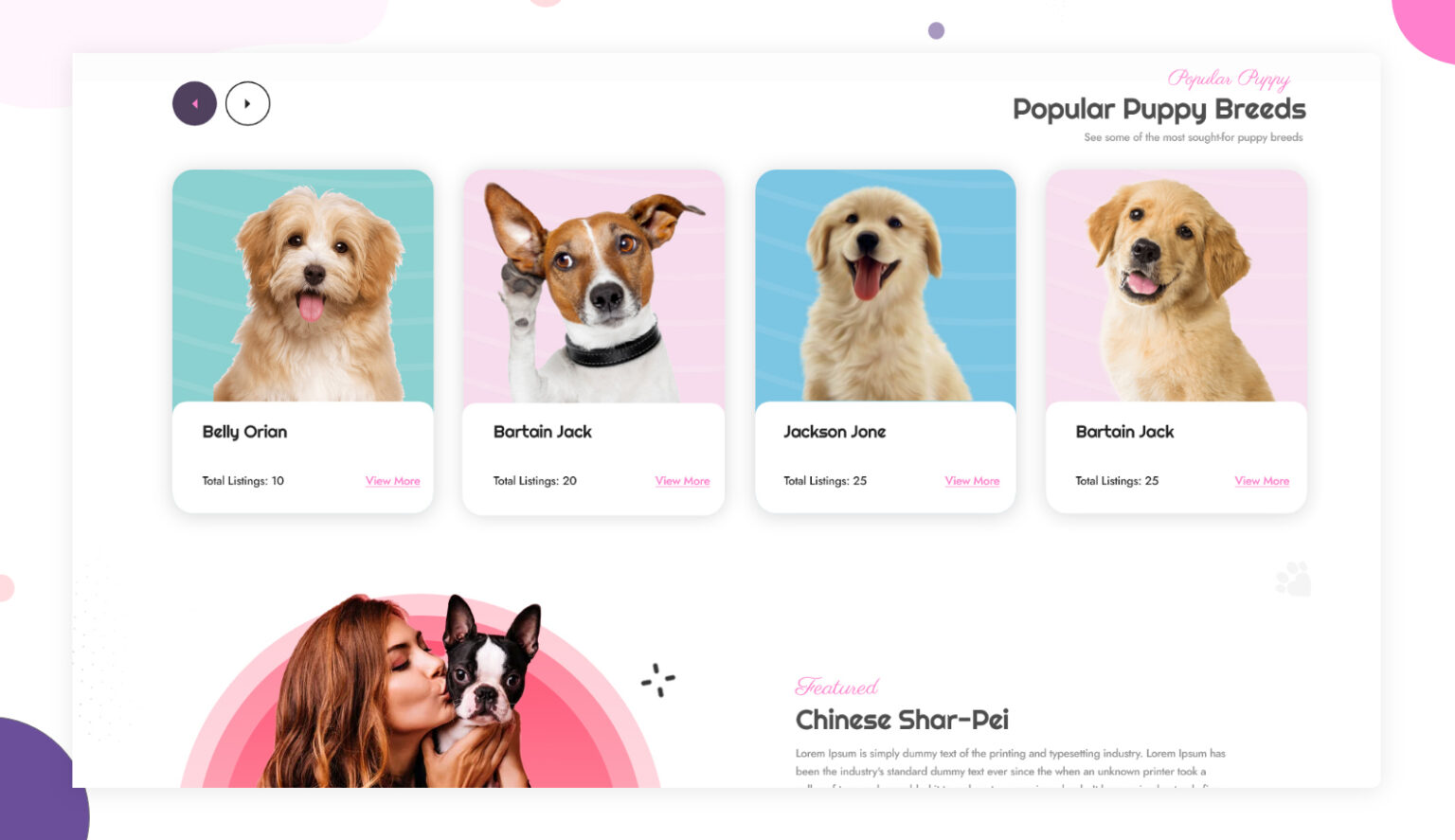Screenshot of a dog information website with a predominantly white background. The design features a half purple circle in the bottom left and the edge of a pink circle in the bottom right, creating a framing effect. In the top right corner, "Popular Puppy Breeds" is written in a bold gray font. The center of the screenshot showcases images of four dogs, each in its own rectangular frame, arranged symmetrically.

1. The first dog is a "Belly Orion," a white fluffy breed, with the text "Total Listings: 10" below it.
2. The second dog is a "Borton Jack," characterized by its white fur and brown head and ears.
3. The third rectangular frame contains "Jackson Joan," set against a blue background, showcasing a fluffy golden-colored dog.
4. The fourth frame features another "Borton Jack," resembling a golden retriever with golden fur, a black nose, and black eyes.

At the bottom part of the webpage, there is an image of a woman kissing a dog. The dog appears to be a French Bulldog, black with a white stripe down the middle of its face, a dark nose, and tall pointy ears. The woman, who is Hispanic with reddish-brown hair and a well-made-up appearance, is holding the dog and affectionately kissing it on the cheek. This section of the page has a pink background. On the right side, the text "Chinese Shar-Pei" is visible.